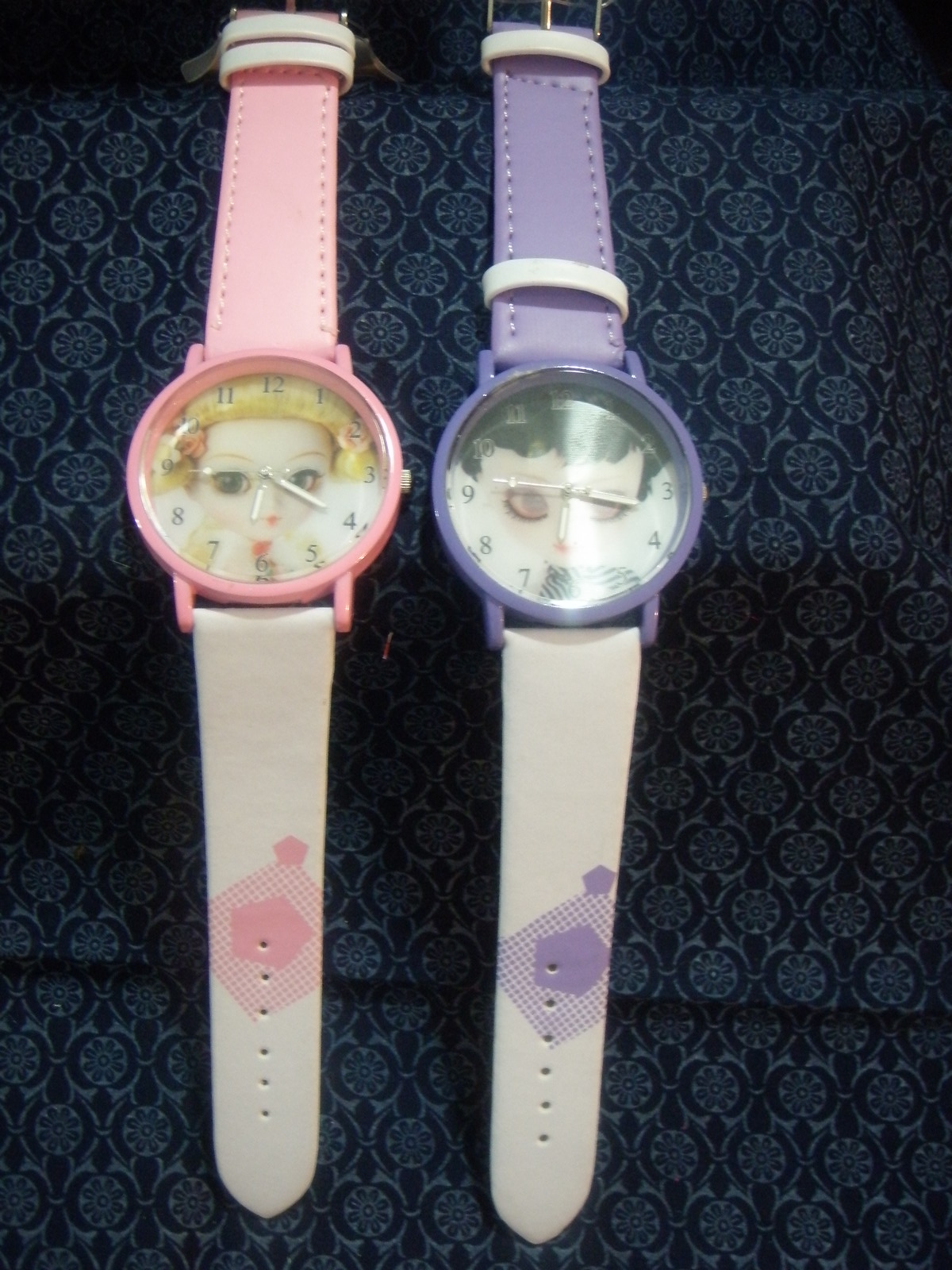The image captures a close-up of two children's watches displayed side by side on a dark, deep blue background featuring a floral motif. The watch on the left has a pink metal fascia, complemented by a pink upper strap and a white lower strap adorned with pink geometric shapes. Its dial showcases a face resembling a geisha or anime character with blonde hair. This watch is set to 6:20. The watch on the right is identical in design but features a purple metal fascia, a purple upper strap, and a white lower strap with purple geometric shapes. The face on this watch depicts a girl with black hair, possibly another anime character. This watch is set to around 6:16. Both watches have two white loops on their respective straps, with the pink watch's loops positioned at the top, while the purple watch has one loop at the top and one near the metal fascia. The floral-patterned background, resembling a blue carpet or paisley shirt, serves merely as a backdrop, drawing all focus to the colorful and detailed watches.